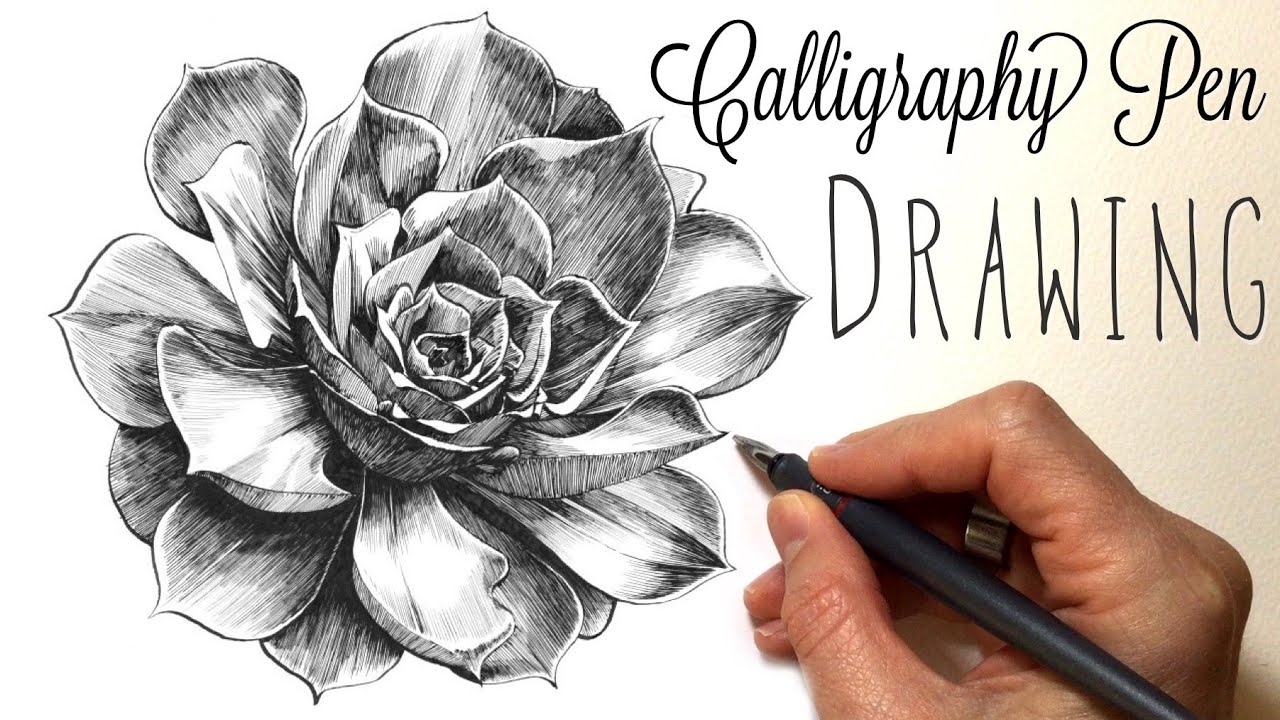The image is an artistic composition featuring both a photograph and a drawing on a white background. Dominating the left side of the image is a highly detailed, hand-drawn flower with numerous layers of petals, which appear to be blooming. The drawing, created with pencil, ink, or pen, showcases larger outer petals and smaller inner petals, adding to its intricate realism with notable shading and light effects.

On the right side of the image, the words "calligraphy pen" are elegantly written in black cursive text, underneath which "DRAWING" is printed in regular, capitalized letters. Below this text, a real-life hand emerges from the lower part of the image. The hand, exposing the top of the fingers and the palm, holds a sleek black pen with a silver tip, typical of a calligraphy pen, poised just to the right of one of the flower's petals.

The interplay of the photographic element and the drawing, coupled with the clean white background and neat calligraphy, creates a visually engaging and cohesive image.